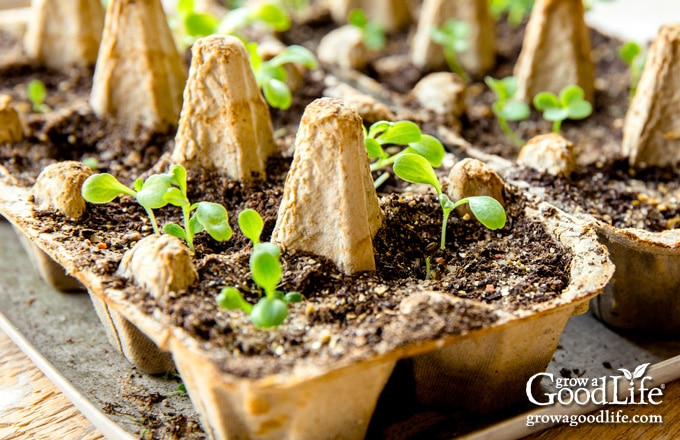This photograph captures a neatly arranged propagation setup using egg cartons to nurture young seedlings. Viewed from above at an angle, the setup comprises brown egg cartons placed on a silver baking pan, which is set atop a blonde wooden surface. Each section of the egg cartons is filled with soil from which vibrant green seedlings are emerging, each with two to three leaves, indicating they have just germinated. The moist soil supports the robust development of these tiny plants. The scene suggests multiple rows of these cartons, as one carton is clearly visible with another beside it. In the bottom right corner of the image, the logo "Grow a Good Life" is visible, with leaves sprouting out of the 'I' in "Life" and the accompanying URL, growagoodlife.com, all rendered in white font, indicating the company likely promoting this effective, eco-friendly method of seed starting.